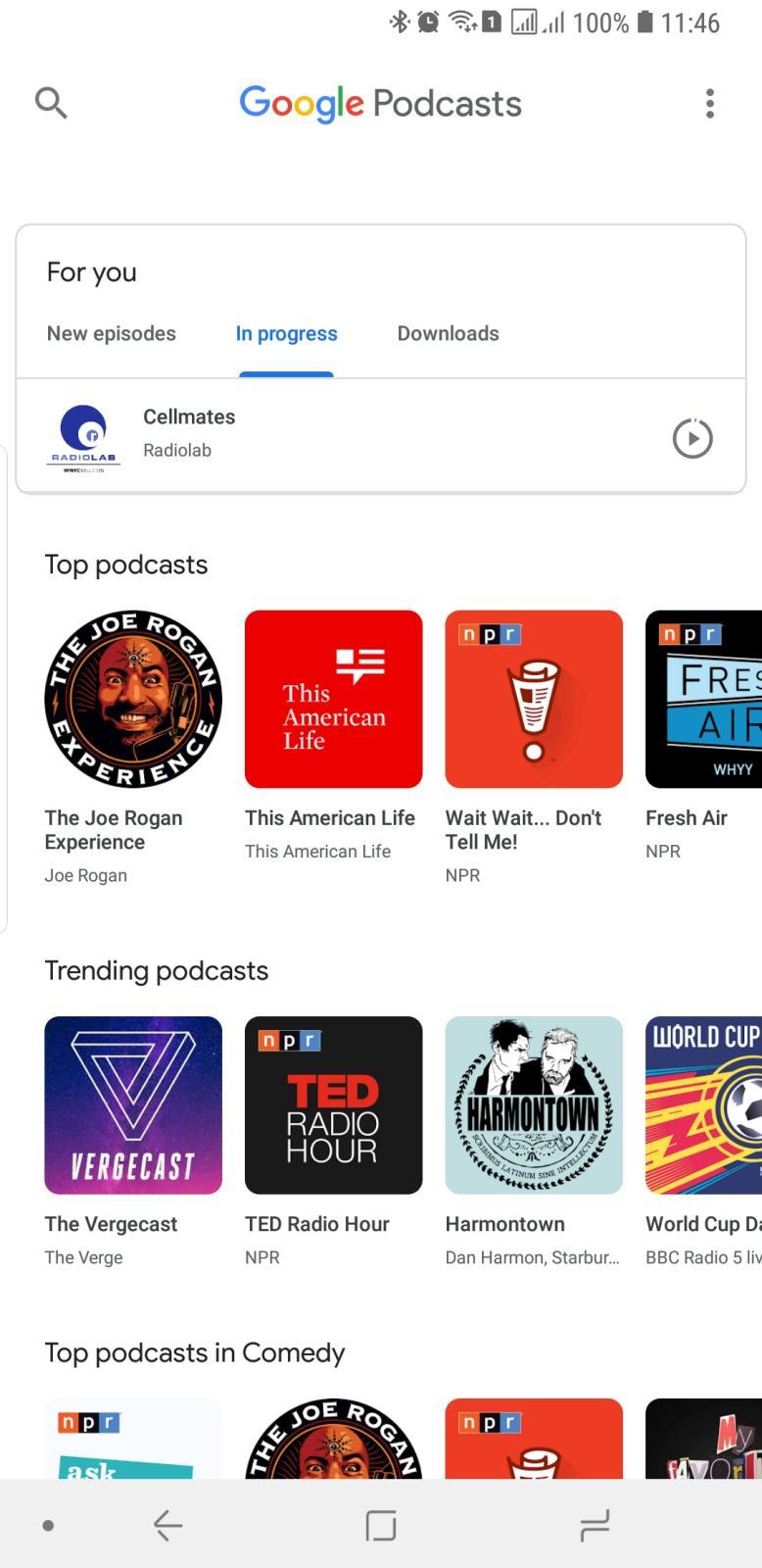This screenshot, captured at 11:46 AM from an Android device, showcases a personalized page on Google Podcasts, evident from the "For You" tab at the top. The user appears to be in the process of downloading or streaming a podcast, as indicated by the progress bar. The top section features a curated list of popular podcasts: "The Joe Rogan Experience," "This American Life," "Wait Wait... Don't Tell Me!," and "Fresh Air," respectively. Below, there are sections for trending podcasts and the top podcasts in the comedy genre. The device’s status bar shows Bluetooth is enabled, the alarm is set, Wi-Fi is in use, and the mobile signal is strong. At the bottom of the screen, navigation icons are displayed: a back arrow on the left, a square icon, likely for home, in the center, and an unidentifiable icon on the right.